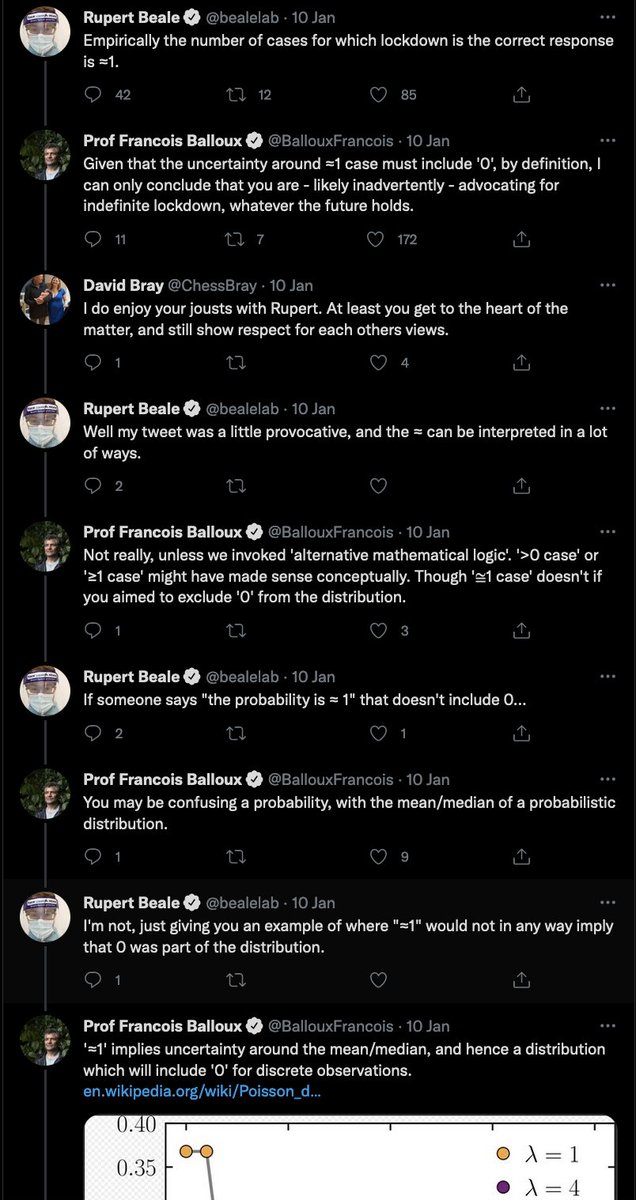**Detailed Caption:**

The image depicts a Twitter conversation between verified users Rupert Beale and Professor Francois Balloux, with their respective Twitter handles @BealeLab and @BallouxFrancois. The original tweet by Rupert Beale, posted on January 10th, reads: "Empirically, the number of cases for which lockdown is the correct response is exactly one." This tweet, featuring Beale's icon, gathered significant interaction, with 42 comments, 12 retweets, and 85 likes.

Professor Francois Balloux responded to Beale's tweet: "Given that the uncertainty around the number one case may and must include zero by definition, I can only conclude that you are likely inadvertently advocating for infinite lockdown whatever the future holds." Balloux's response further ignited the conversation, resulting in 11 comments, 7 retweets, and 172 likes.

The discussion extends as David Gray joins, followed by a back-and-forth exchange between Rupert Beale and Professor Francois Balloux, punctuating their debate with additional comments. At one point, Balloux concludes his argument by sharing a Wikipedia link, albeit the image of this link has been cut off, leaving the concluding context incomplete.